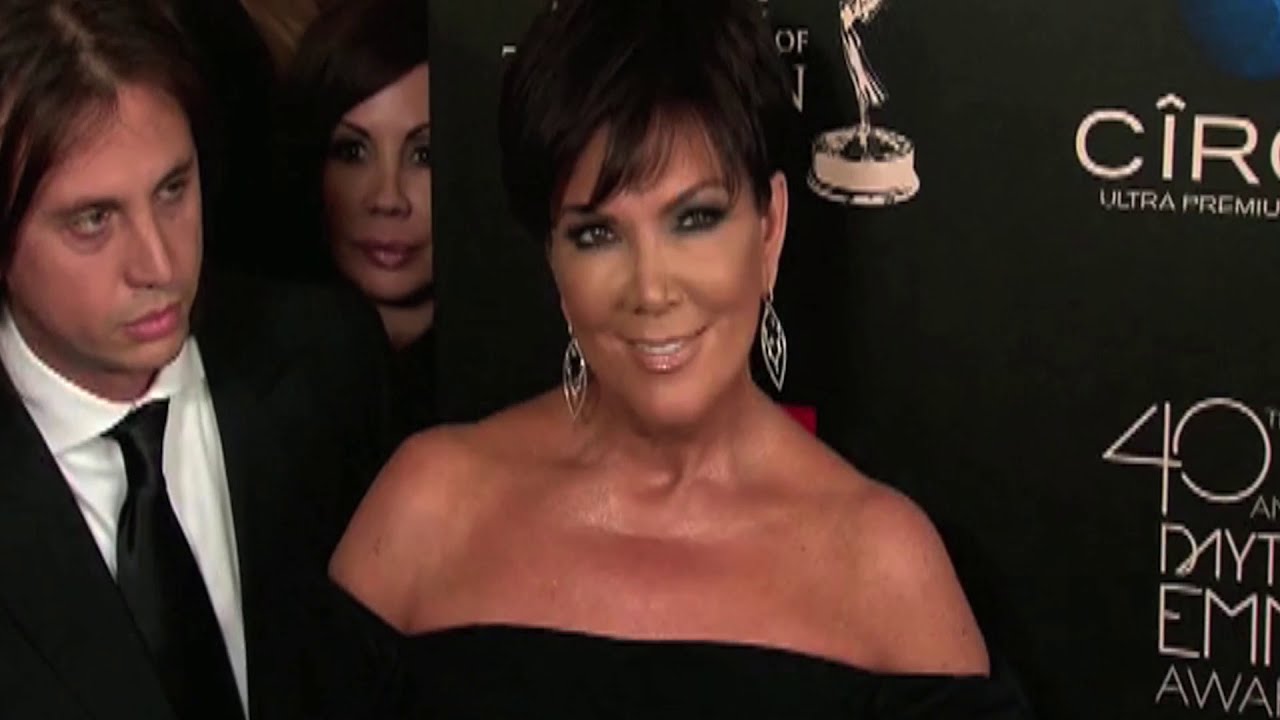This image captures Kris Jenner at the 40th Annual Daytime Emmy Awards. Positioned center stage, Kris Jenner is elegantly dressed in an off-the-shoulder, low-cut black dress, accentuated with large silver earrings and prominent eyeshadow. Her short dark hair frames her face as she smiles warmly in front of a partially visible black backdrop displaying the text "CIRC, Ultra Premium, 40th Annual Daytime Emmy Awards." To her left stands a younger man with shaggy brown hair, sporting a black jacket, white shirt, and a tie, who appears somewhat confused as he looks in her direction. In the background, another woman with dark hair, pink lipstick, and subtle eyeshadow can be seen, partially obscured in shadow, adding depth to the composition.